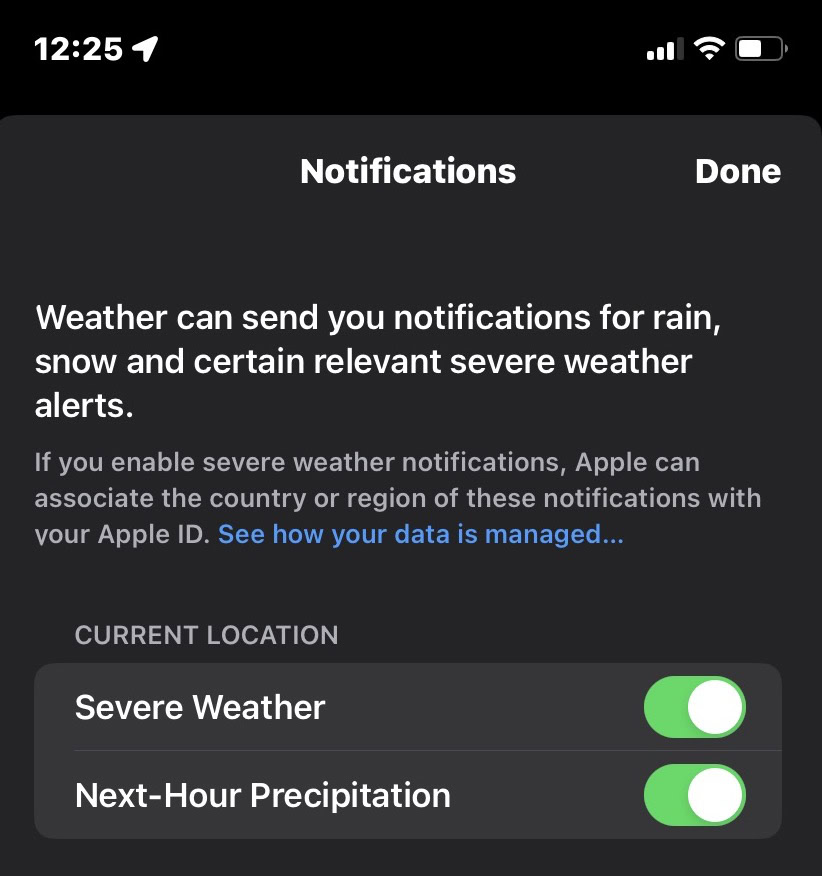This image is a cropped screenshot of a cell phone's notification settings tab, specifically focused on weather notifications. The top portion of the screen displays the current time in the top left corner along with a location icon indicating that location services are enabled. In the top right corner, icons for Wi-Fi strength, cellular signal strength, and battery percentage are visible.

The main content area is a notification settings screen set against a dark background. Centered at the top is the word "Notifications" in white text, with a "Done" button positioned to the right. Below this, the section details continued notifications for weather, including alerts for rain, snow, and certain severe weather conditions.

A light gray informational text beneath provides additional context: "If you enable severe weather notifications, Apple can associate the country or region of these notifications with your Apple ID." There is also a blue link labeled "See how your data is managed."

Following this, the section offers customizable options. The first option, labeled "Severe Weather," has a green toggle switch indicating it is currently enabled. The second option, "Next Hour Precipitation," also has an active green toggle switch. The toggles are designed with a green background, affirming their enabled status.